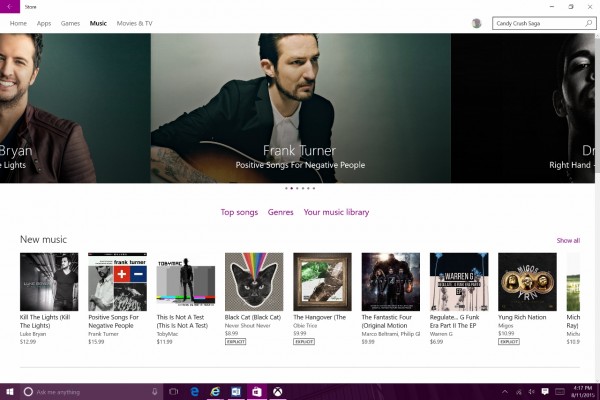The image appears to be a screen capture from an entertainment website, predominantly featuring a music section. The background is predominantly white, creating a clean and minimalistic layout. 

At the very top, on the left-hand side, there is a purple button situated next to the word "store," suggesting an interactive element for users, potentially leading to the website's store section. On the right-hand side of the top bar, a search box is visible with the query "Candy Crush Saga” typed in, likely indicating the user’s next intended search. Above the search box, there are three icons, including an 'X' for closing the search box and two unidentified icons.

Central to the image is a large composite shot featuring three different musicians. The most prominent image in the center showcases Frank Turner, with text detailing his album "Positive Songs for Negative People." On the left, although partially obscured, the name Luke Bryan is identifiable along with an image hinting at his performer persona. The right side features an individual whose name appears to begin with 'D,' speculated to be Drake, but the image is cut off, omitting the song titles.

Below this composite image, the background remains white, displaying headings such as "Top Songs," "Genres," and "Your Music Library." Alongside these headings are navigation dots indicating a carousel or slider feature for viewing additional content. Under the main composite image, there is a section labeled "New Music," showcasing thumbnails of eight different songs or albums, including entries from Frank Turner and Toby Mac.

At the very bottom of the screen, the image cuts off, showing what appears to be the bottom part of a desktop interface. Menu choices line the top of the page, including "Home," "Apps," "Games," "Music," "Movies," and "TV," with "Music" highlighted in a darker color, signifying active selection. This results in the current page displaying music-related content exclusively.